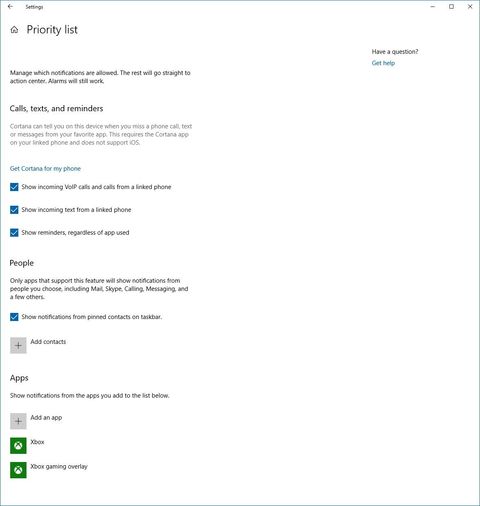The image is a screenshot of a computer screen with a white background. In the top left-hand corner, there are icons for settings and a back button. In the top right-hand corner, there are icons for minimizing, maximizing, and closing the screen. Below the settings icon on the left side is a house icon labeled "Priority list."

Toward the right side, there's a prompt reading "Have a question?" followed by a blue "Get help" text link. Beneath "Priority list," a heading states, "Manage which notifications are allowed. The rest will go straight to the action center. Alarms will still work."

Further down, there's a section titled "Calls, texts, and reminders." The description reads, "Cortana can tell you on this device when you miss a phone call, text, or message from your favorite app. This requires the Cortana app on your linked phone and does not support iOS." 

A blue link labeled "Get Cortana for my phone" follows this description. Below this link, there are three checkmark boxes with the following options:
1. "Show incoming VOIP calls and calls from a linked phone"
2. "Show incoming text from a linked phone"
3. "Show reminders, regardless of app used"

Next is a section titled "People." It notes, "Only apps that support this feature will show notifications from people you choose, including mail, Skype, calling, messaging, and a few others." There is a checked checkbox with the option "Show notifications from pinned contacts on taskbar," followed by an "Add contacts" button.

The section "Apps" follows, stating: "Show notifications from the apps you add to the list below." There is an "Add an app" button. The list includes two entries: "Xbox" and "Xbox Game Bar."